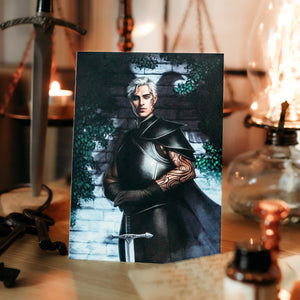This square image features a prominent rectangular poster standing upright on a wooden surface, possibly a desk or a counter. The poster depicts a man dressed in black armor, with elaborate tattoos visible on his uncovered arms and black gloves adorning his hands. He holds a sword in front of him, its black handle firmly gripped while its silver blade points downward. The man has short, whitish-yellow hair and stands against a brick wall background that transitions from white at the bottom to black at the top. Ivy and green leaves trail down from the top and both sides of the wall, adding a touch of organic detail. The setting around the poster includes a chain hanging from the wall, likely supporting potted plants, and an oil lamp to the right. A small glass bottle with a black cap is visible in the lower right corner, and another sword appears to be embedded in a piece of wood from the upper left. The background, although somewhat blurred, also suggests additional elements like weights and measures, bulbs, and flames, contributing to a slightly chaotic yet intriguing scene.